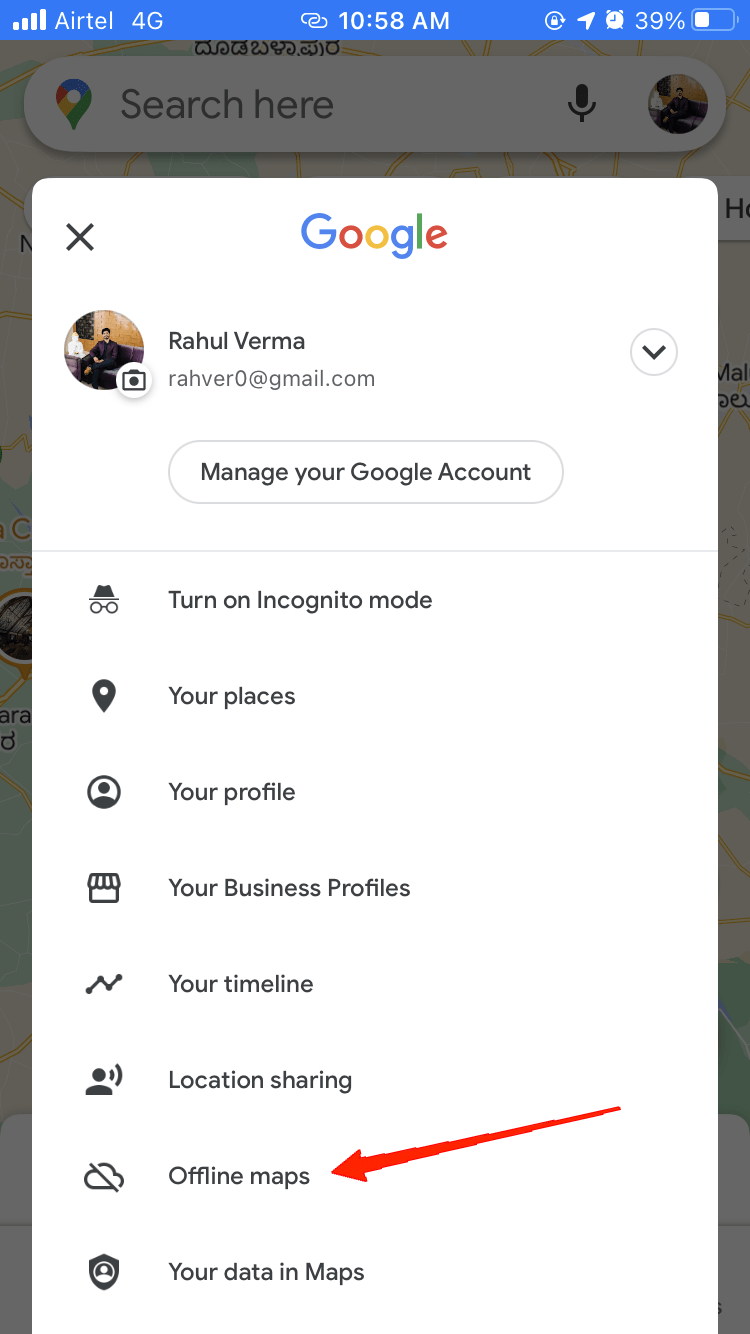Screenshot of a smartphone displaying the Google Maps "Your Profile" screen. At the top, a blue status bar shows full signal strength with "Airtel 4G" written in white text, along with the current time "10:58 a.m.", a lock symbol, GPS indicator, alarm clock icon, and a battery life at 39%, which is less than half full.

The background of the screen is grayish with the black text "Search here in Maps." At the top left, there is a black "X" to close the screen. The Google logo is visible below that. In the center, there's a profile picture of a person named "Rahul Verma" along with his email address, which should have been obscured for privacy.

Below the profile details, several options are listed: "Turn on in commuter mode," "Your places," "Your profile," "Your business profiles," "Your timeline," "Location sharing," "Offline maps," and "Your data in Maps." A prominent red arrow points towards "Offline maps," suggesting the screenshot is part of an instructional guide on accessing offline maps when without cellular or Wi-Fi service.